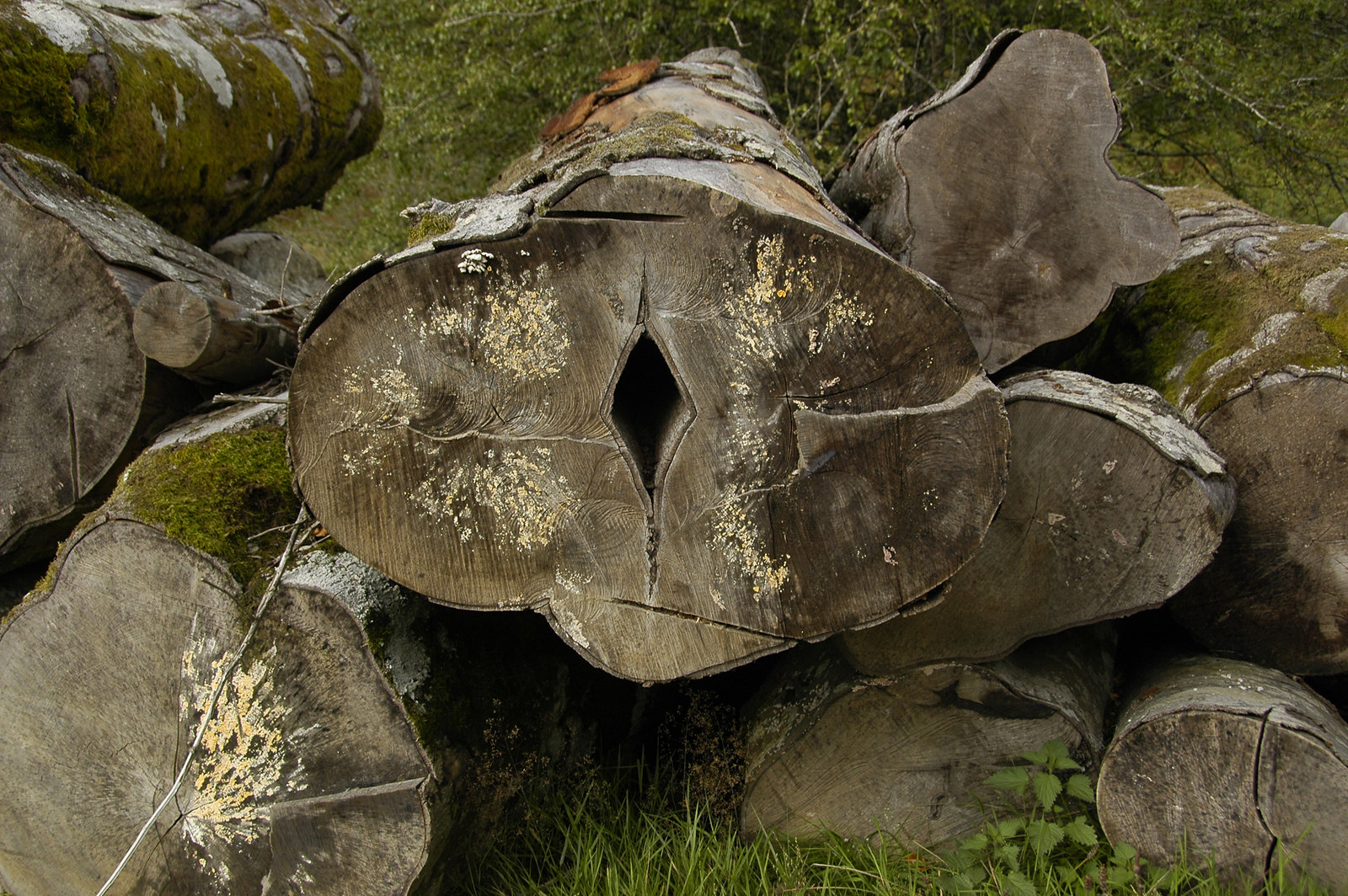This detailed photograph showcases multiple logs stacked on top of one another, revealing their smooth, tool-cut cross sections. The aged logs display signs of forest growth, with moss and dead leaves replacing much of their missing bark. The logs, irregularly shaped and more oval than round, lie horizontally on the ground with grass peeking out from underneath. Central in the image is a distinctive log with a natural diamond-shaped hole running through its center. This log, like its counterparts, also features some tan or white discoloration on its flat cut surface, along with patches of yellow growth. Surrounding this central log, we can observe five logs to the right and three logs, along with a smaller branch, to the left—several of which are enveloped in moss. In the background, a mix of brush and shrubs further sets the scene within a forest setting.